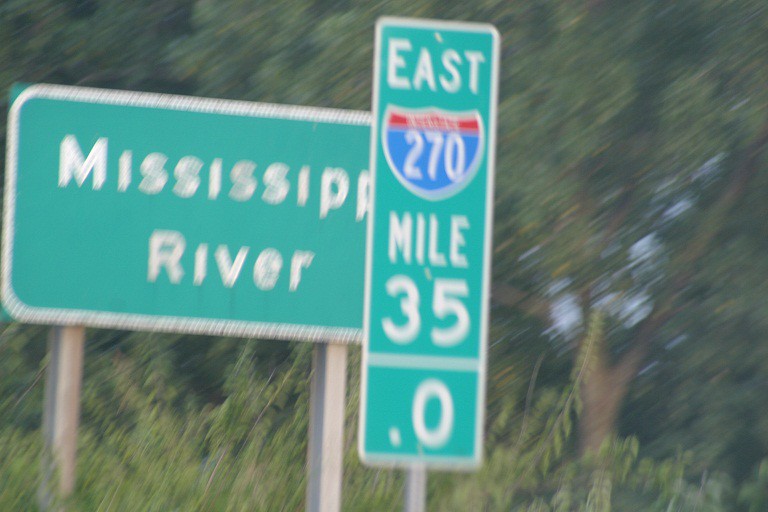In the foreground of the image, a tall, vertical teal sign displays "East Interstate 270, Mile 35.0" in white lettering. Positioned behind it is a larger, horizontally oriented sign, also teal with white text, that reads "Mississippi River." The scene features a forested background with trees, giving the image a natural, woodland setting. A slight blur effects the image, yet the signage remains legible, suggesting the photo was taken along an interstate route.